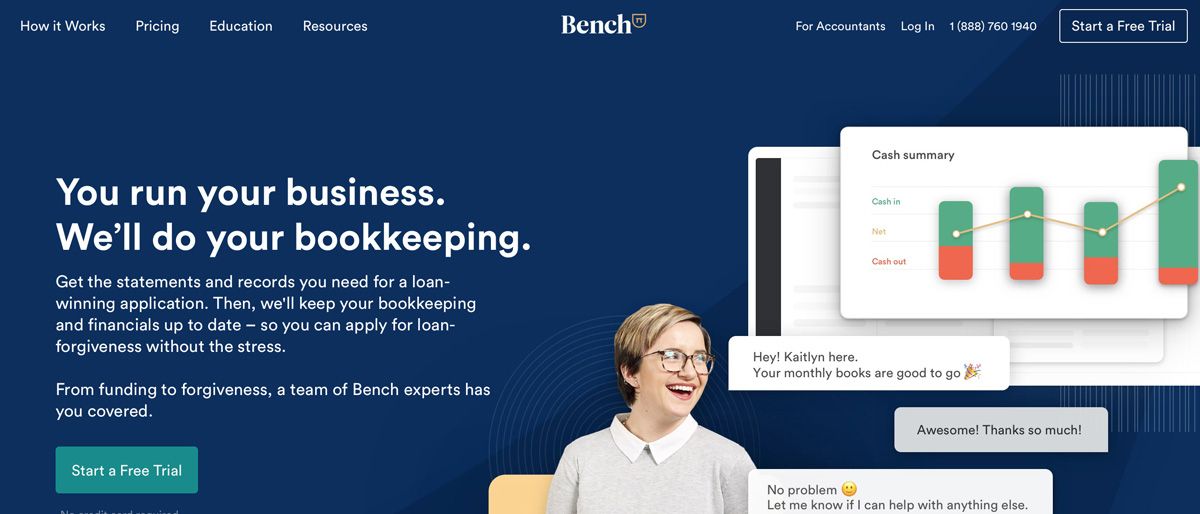The image is a screenshot taken from the Bench website. Dominating the center of the image, the website name "Bench" is prominently displayed. The background is a deep navy blue, providing contrast to the white text in the navigation bar at the top. This bar features clickable areas labeled "How It Works," "Pricing," "Education," "Resources," and extending further to the right, it includes options for "For Accountants," "Log In," and a phone number, "1-888-760-1940." A distinct "Start a Free Trial" button is positioned here as well.

On the right side of the page, a cash summary with various informational boxes is visible. Toward the bottom center, a smiling woman—presumably named Caitlin—is pictured with a speech bubble stating, "Hey Caitlin here, your monthly books are good to go." A respondent's message reads, "Awesome, thanks so much," to which Caitlin replies, "No problem, let me know if I can help with anything else."

To the left, the bold text reads, "You run your business, we'll do your bookkeeping," followed by a descriptive paragraph detailing this offer. Nearby, another "Start a Free Trial" button is highlighted in a bluish-green box.